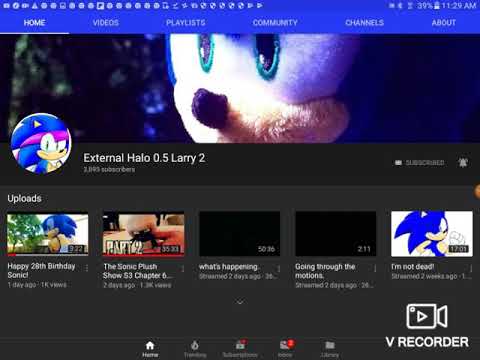The image displays a blurry screenshot of a video platform that resembles YouTube yet appears to be a knockoff version. The interface includes a bottom menu with five options: Home, Trending, and three unreadable icons. The top section features a Sonic the Hedgehog plush toy image as the header profile and displays categories like Home, Videos, Playlists, Community, Channels, and About on a blue header bar. The profile name displayed is "Eternal.Halo 0.5 Larry 2" and the profile picture is also of Sonic the Hedgehog. The uploaded content, indicated by at least five videos, seems to be entirely focused on Sonic the Hedgehog, with a specific mention of celebrating Sonic's 28th birthday. The border of the screen has an extensive number of icons, approximately 25-30 on the left and a 39% battery indicator on the right, suggesting the device might be a laptop rather than a phone. The image leaves many details unclear and presents a somewhat confusing array of icons and information.